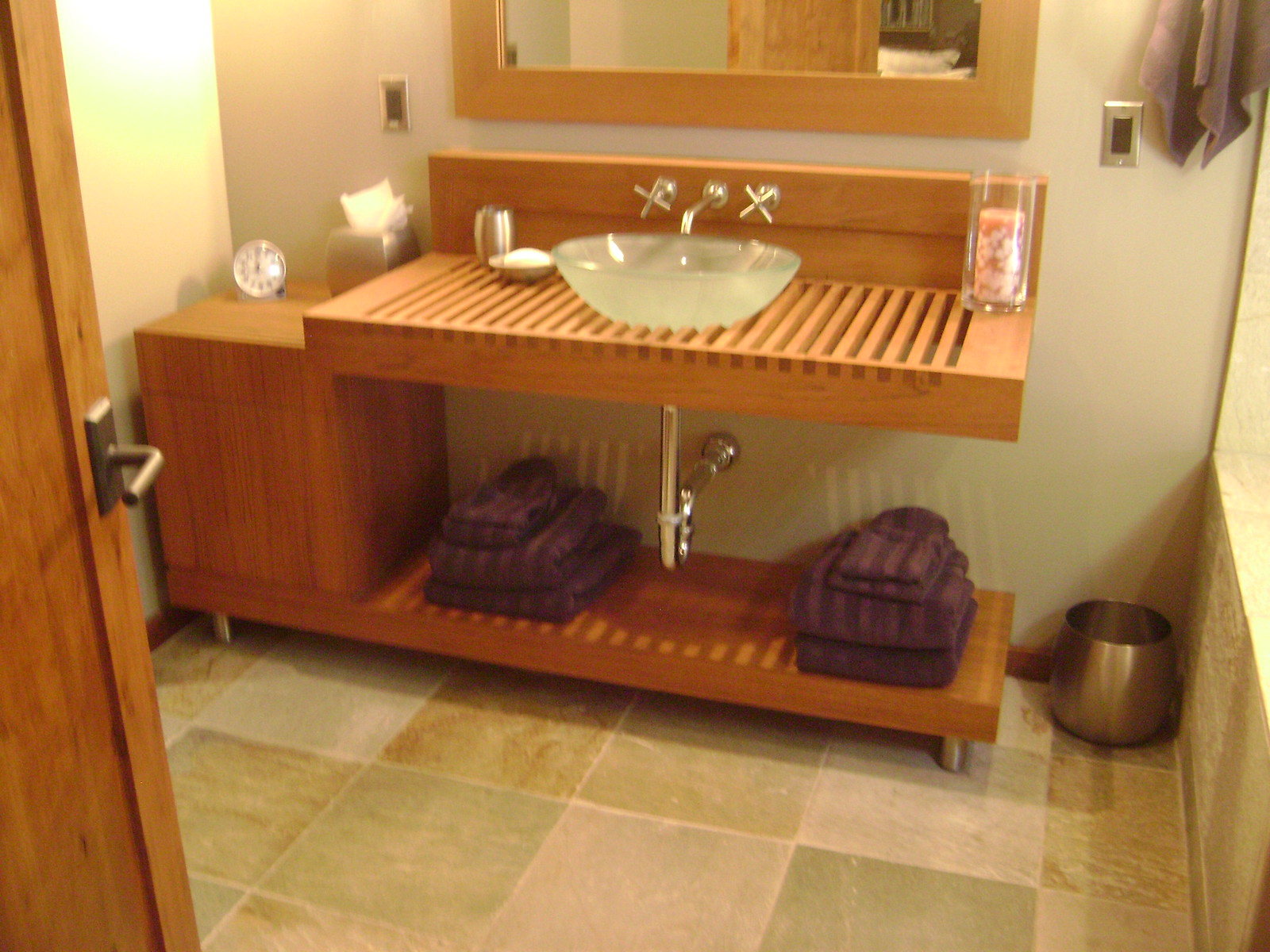This image, taken from the doorway of a home restroom, captures the serene and organized sink area. The sink rests atop a bamboo-like wooden countertop, with a matching shelf below and an adjacent wooden counter. The sink itself is a striking large glass bowl, complemented by three wall-mounted spigot controls: two on either side for hot and cold water, and a central spout for water flow. To the right of the countertop, a large white candle in a glass jar adds a touch of ambiance. On the left, a chrome napkin holder and a clock provide both practicality and style. Below the sink, neatly folded purple towels are stacked on either side on the wooden shelf. The floor is tiled with large, square tiles featuring an array of earthy tones, contributing to the bathroom's warm and natural aesthetic.